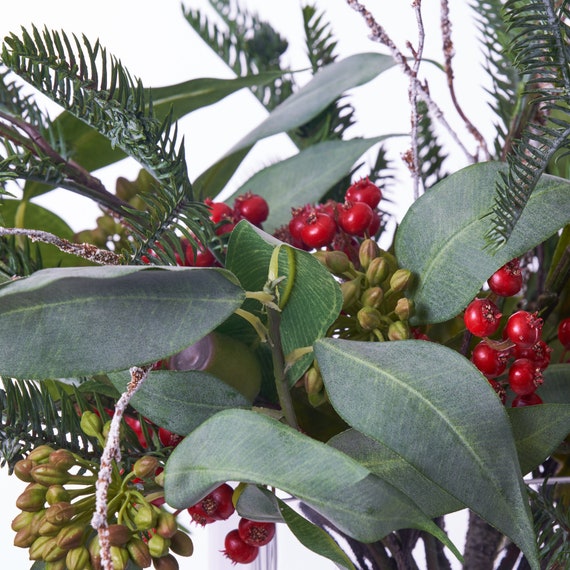The image is a bright, well-lit square image with a plain white background, showcasing a detailed close-up of a Christmas-themed plant arrangement. The composition includes realistic-looking decorative elements that could be mistaken for real flora. Central to the arrangement are clusters of vibrant red holly berries and green eucalyptus seeds with brown tips, some of which appear as unopened flower buds. Accompanying these are an assortment of leaves: large, solid, and pale green leaves dusted with a white powder, smaller line-like leaves forming compound structures, and pine needles flanking both sides of the arrangement. The greenery and festive elements create a natural yet decorative Christmas scene.